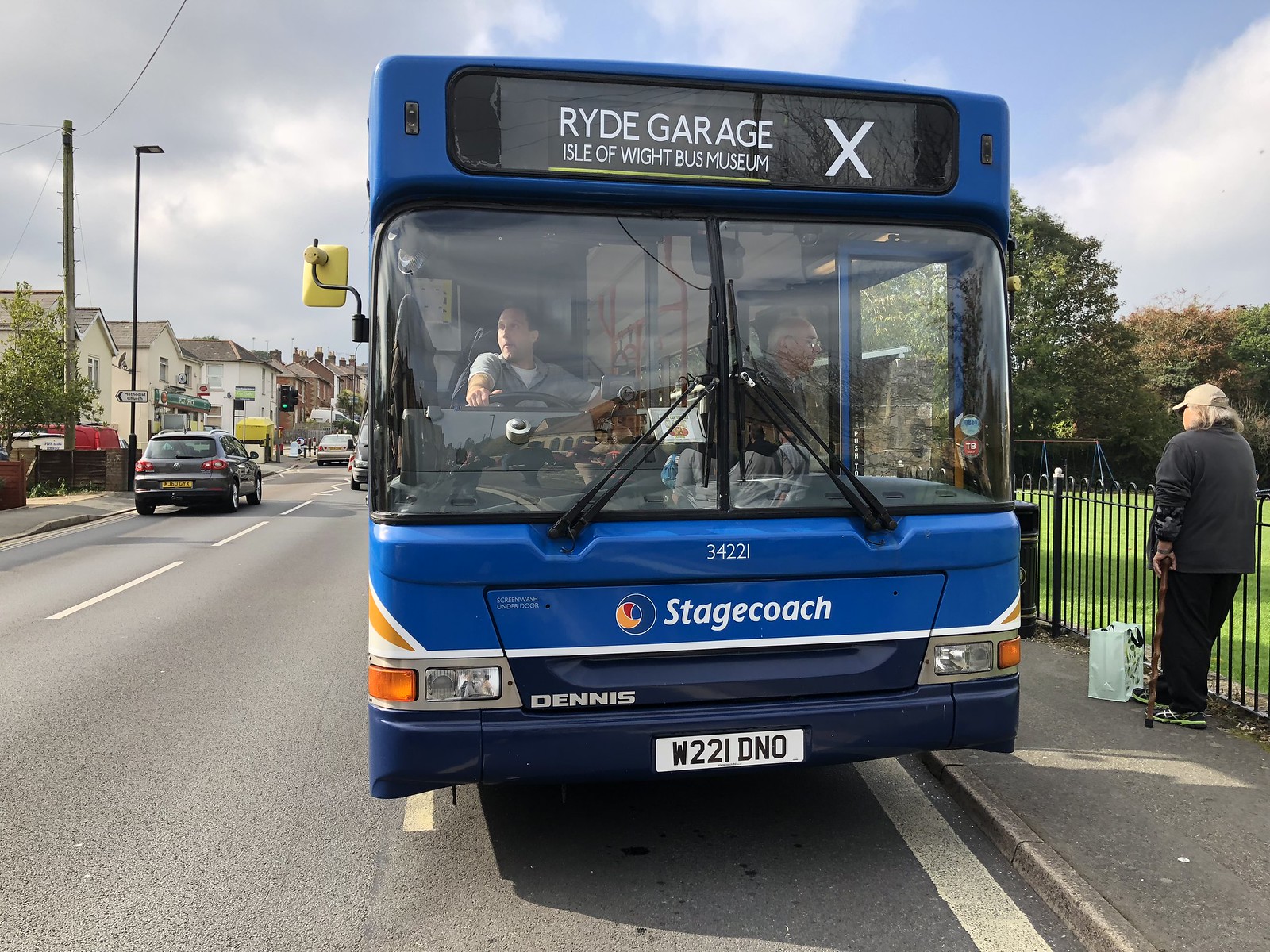A blue bus, prominently displaying "Stagecoach" in white letters on the front, is parked along a city street. The license plate reads W221DN0 and the bus is identified as number 34221. Above, it features the inscription "Ride Garage, Isle of Wight Bus Museum," accompanied by a white X. The driver, visible through the windshield, is dressed in a short-sleeve gray shirt. The bus doors are open, and an elderly man with white hair, glasses, and a dark coat is alighting. On the right side of the pavement, a man with a ball cap stands by a black wrought iron fence, holding a cane. At his feet is a white tote bag. The street scene includes several cars driving in the opposite direction, against a backdrop of buildings and a partly cloudy sky.